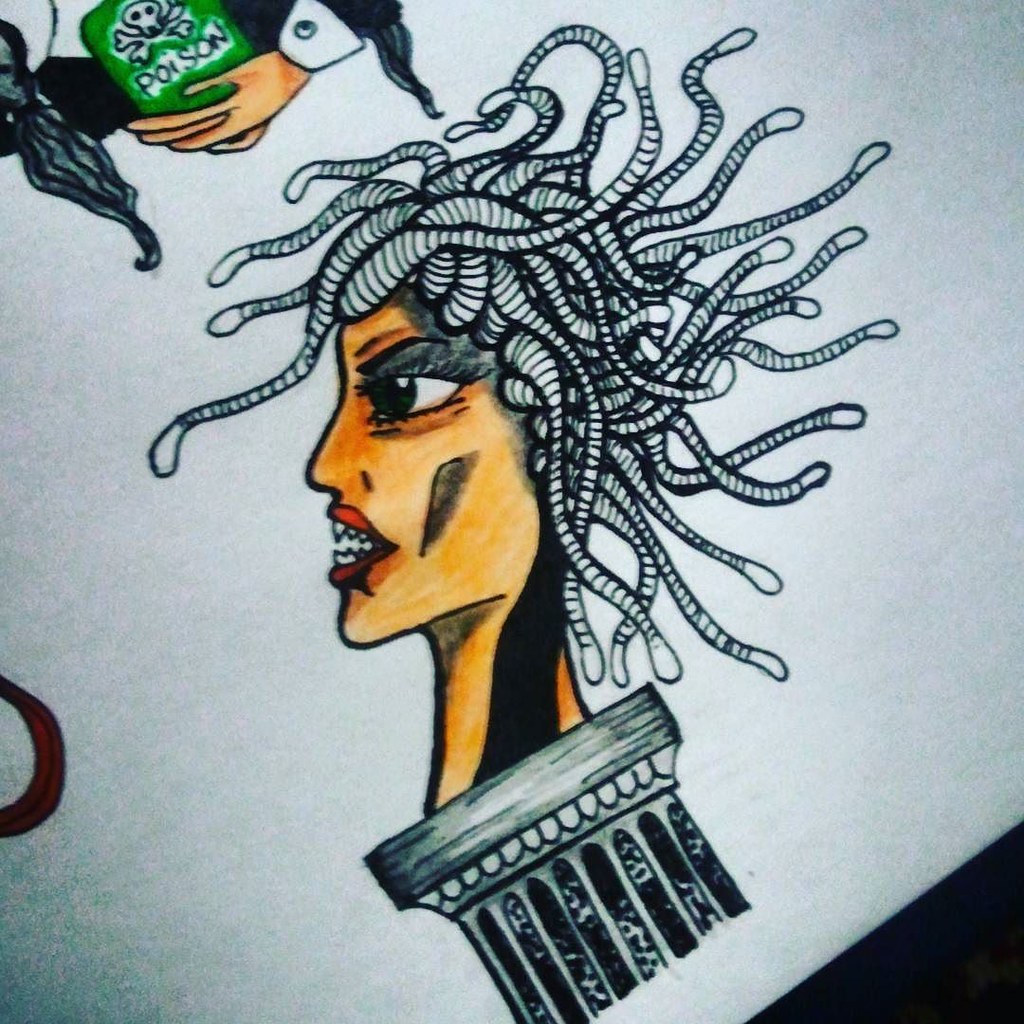This image features a meticulously crafted drawing on a white sheet of paper, rendered in black ink and enlivened with colored pencil or marker. Starting from the upper left corner, a Caucasian hand, detailed with realistic shading, grasps a vividly green bottle labeled "Poison" alongside a menacing skull and crossbones. From the hand dangle two hairy-looking protrusions, adding an unsettling detail. Below, in the center and serving as the focal point of the composition, is a striking profile of a Medusa-like head. However, diverging from traditional mythology, her hair is composed of writhing worms rather than snakes, contributing to an eerie and captivating visage. Her sharp, pointy teeth enhance her menacing appearance, and her black eye and flesh-toned lips, which are tinged with a subtle pink, provide further depth and intrigue. The entire figure is mounted on a pedestal, grounding the fantastical image in a position of prominence.